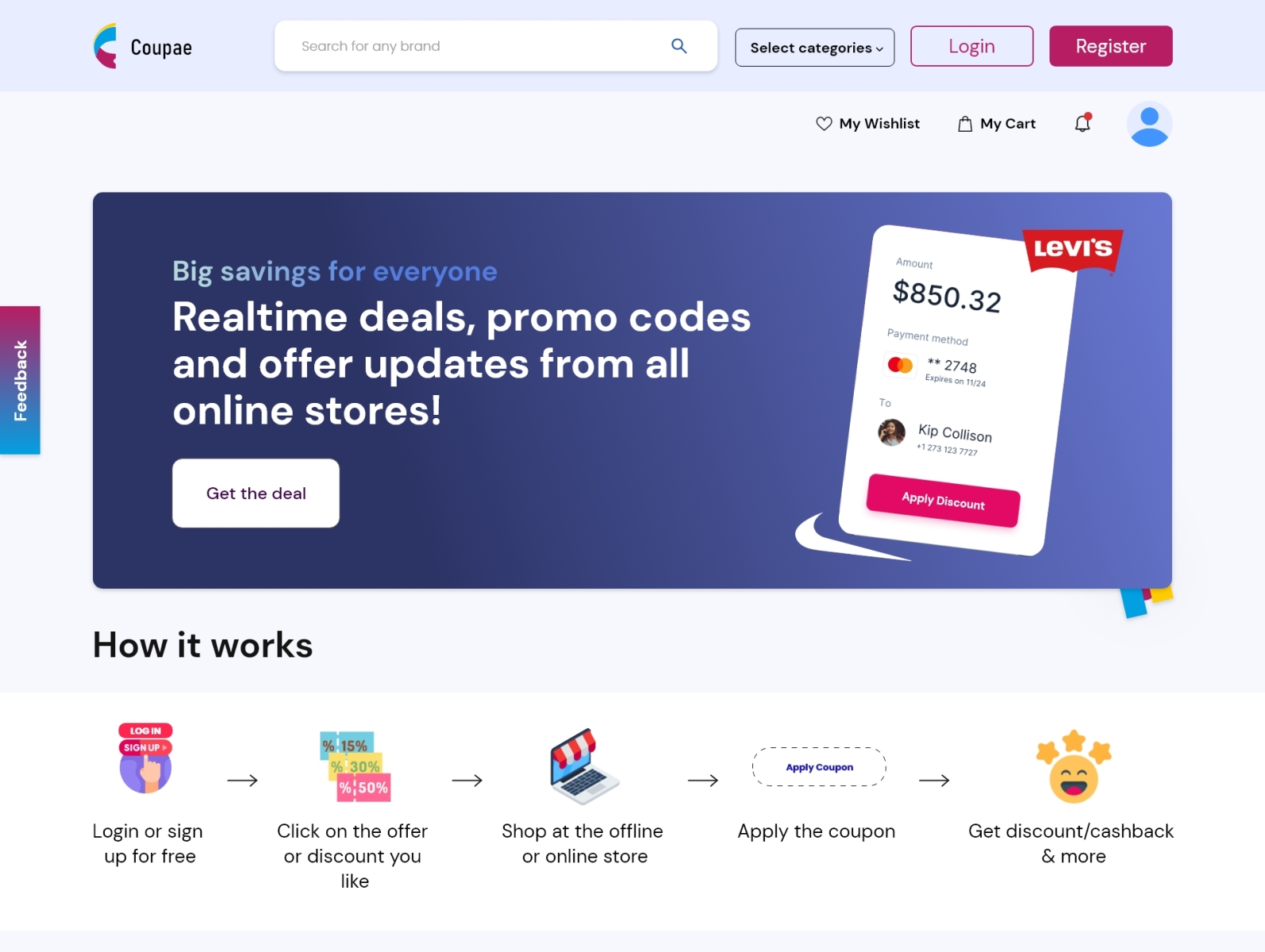The screenshot depicts a clean and user-friendly interface of a shopping website, possibly a pop-up window associated with it. The top of the page features a gray rectangle displaying the website's name, "Coupe," accompanied by a half-circle blue and magenta "C" logo. Adjacent to the logo are a white search bar, a category drop-down menu, and log-in and register buttons. The register button stands out in magenta with white text.

At the bottom of the screenshot is a section titled "How it works," illustrated with arrows guiding the user through the process, moving from left to right. It outlines the steps: log in or sign up (illustrated by a hand pressing a sign-up button), select an offer or discount, shop at an offline or online store, apply the coupon, and finally, receive discounts and cashback rewards, represented by a large smiley face surrounded by stars.

Positioned centrally is a rectangular advertisement with a blue background and bold text proclaiming "Big Deals for Everyone." This section highlights "real-time deals, promo codes, and offer updates from all online stores." On the right, the advertisement features recognizable logos, including the Nike swoosh and a white angled rectangle with the Levi's logo. Additionally, it displays a payment amount of $850.32 alongside an "Apply Discount" button.

Overall, the website's layout is symmetrical, highly organized, and visually appealing, ensuring ease of navigation for users.